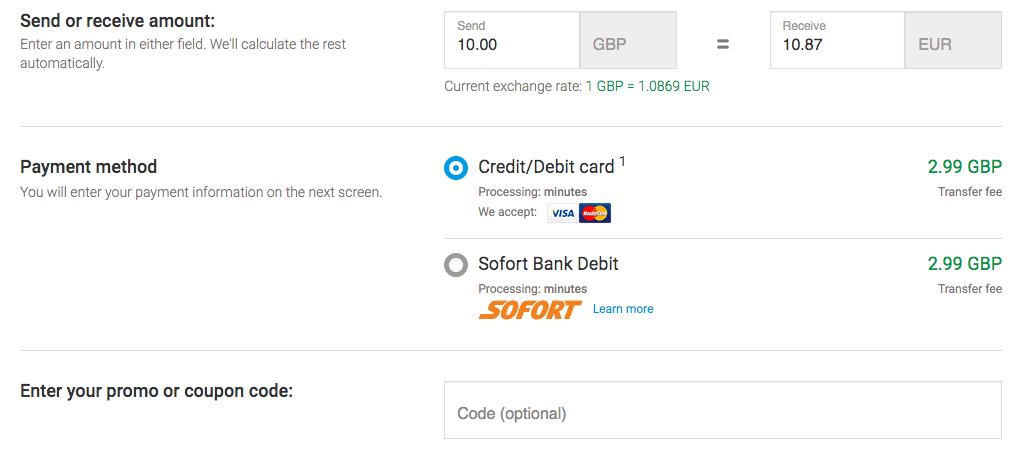The image is a detailed screenshot of a currency conversion website interface. 

In the upper left corner of the screen, a clear black font on a white background displays the message: *"Send or receive amount. Enter an amount in either field, we'll calculate the rest automatically."* To its right, there is a box showing the conversion rate example: *"Send 10 GBP equals receive 10.87 EUR."* Directly below this, the current exchange rate is explained: *"1 GBP equals 1.0869 EUR."*

Further down, a box in the upper left corner is labelled *"Payment Method."* Below this title, in a lighter font, it states: *"You will enter your payment information on the next screen."*

To the right, there are two selectable payment options:

1. The top option is highlighted with a blue bullseye indicating it is selected. It reads *"Credit/Debit Card."* Below this, the text mentions *"Processing time: minutes."* It also notes that both Visa and MasterCard are accepted, with a transfer fee of *"2.99 GBP."*
  
2. The bottom option, which is not selected, is *"Sofort Bank Debit."* It also processes in minutes and has an equivalent transfer fee of *"2.99 GBP."*

Below this section, there is another box labelled *"Enter your promo or coupon code."* An empty, optional input field follows this label, marked *"Code (optional)."*

This comprehensive layout ensures that users can easily understand and navigate through the process of converting and sending money using various payment methods.